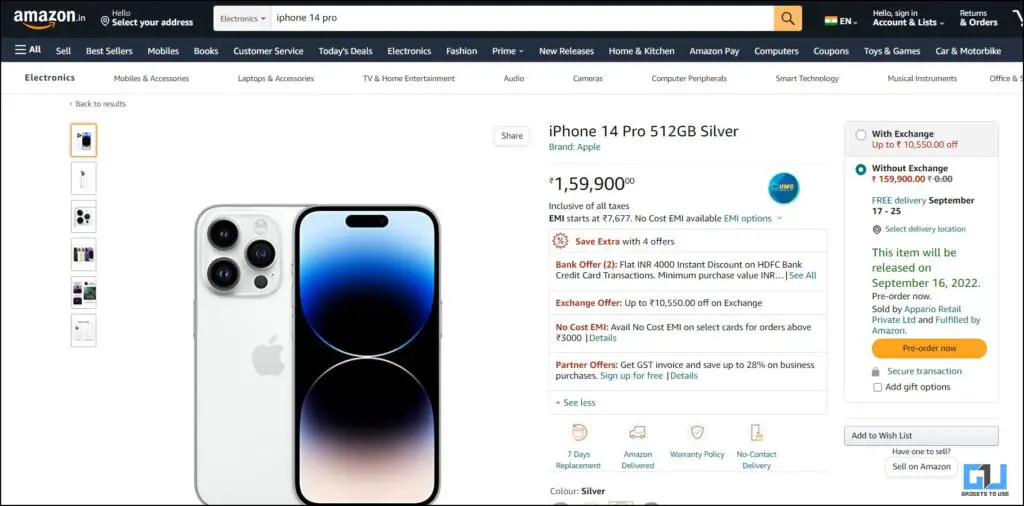Screenshot of an Amazon web page featuring an iPhone 14 Pro with 512GB storage in silver listed for ₹159,900. The iPhone listing, positioned towards the center of the image, includes options for "Without Exchange" and "With Exchange," as well as buttons for delivery options and pre-order.

The top of the web page displays the Amazon home bar, with the Amazon logo situated in the top-left corner. Directly below the logo is a full-width navigation bar containing buttons with white text for various categories, including Amazon Pay, customer service, electronics, fashion, Prime, news releases, and coupons.

In the middle of the top section, a prominent white search bar is visible, accompanied by a yellow search button featuring a black magnifying glass icon. To the right of the search bar, the country indicated is India. Additionally, on the top-right corner, there are buttons for "Sign In" and "Returns & Orders."